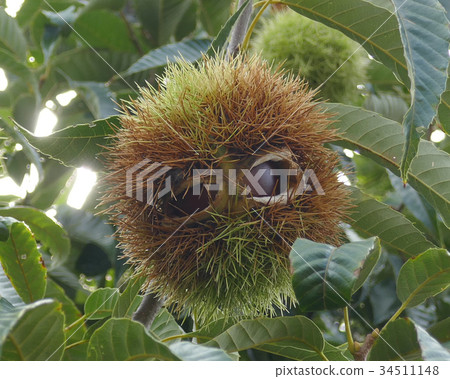This stock photo image features a distinctive natural scene captured in vivid detail. At the very center of the photograph is a circular, prickly, shell-like object resembling a conker, ensconced within a nest of twigs and grass. Surrounding this central focus are numerous large, green leaves that contribute to the lush and exotic setting, suggesting a vibrant outdoor environment far removed from urban life. The photograph's overall color palette prominently features green, brown, and hints of yellow and orange, adding to the natural ambiance. Overlaying the image is a watermark that reads "Pixta" with a diagonal 'X', indicating the stock photo origin. At the very bottom of the image, a white strip with black text states "PixtaStock.com-34511148," likely a code pertinent to the stock photo database.